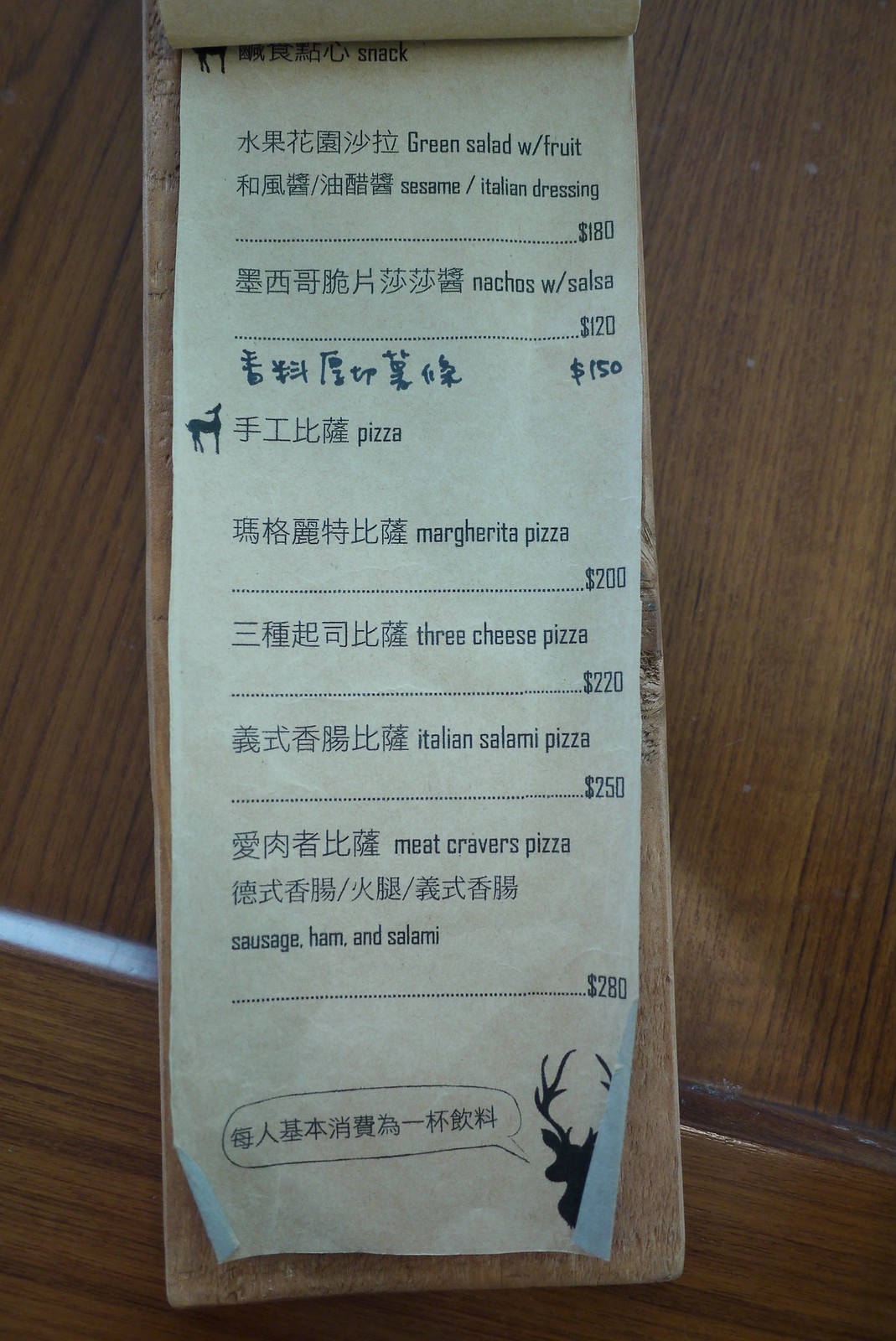The image depicts the menu of a restaurant located in a Southeast Asian country, identifiable by the presence of Asian characters accompanying the English text. The menu features notably high prices, likely reflecting the local currency rather than US dollars. For instance, a "Green Salad with Fruit" offered with either a pesto mix or Italian dressing is priced at $180. Additionally, "Nachos with Salsa" are listed at $120. 

Several pizzas are detailed, including a Margherita Pizza, Three Cheese Pizza, Italian Salami Pizza, and a Meat Cravers Pizza containing sausage, ham, and salami, each priced at $280. The visual also includes the silhouette of a reindeer's head, with a speech bubble containing text in the local Asian script, making it incomprehensible to non-native readers. The menu appears to be part of a larger collection, as visible attached pages suggest more options are available by flipping through the menu. These thin paper-like pages are held together by a slender wooden strip, providing support and organization.